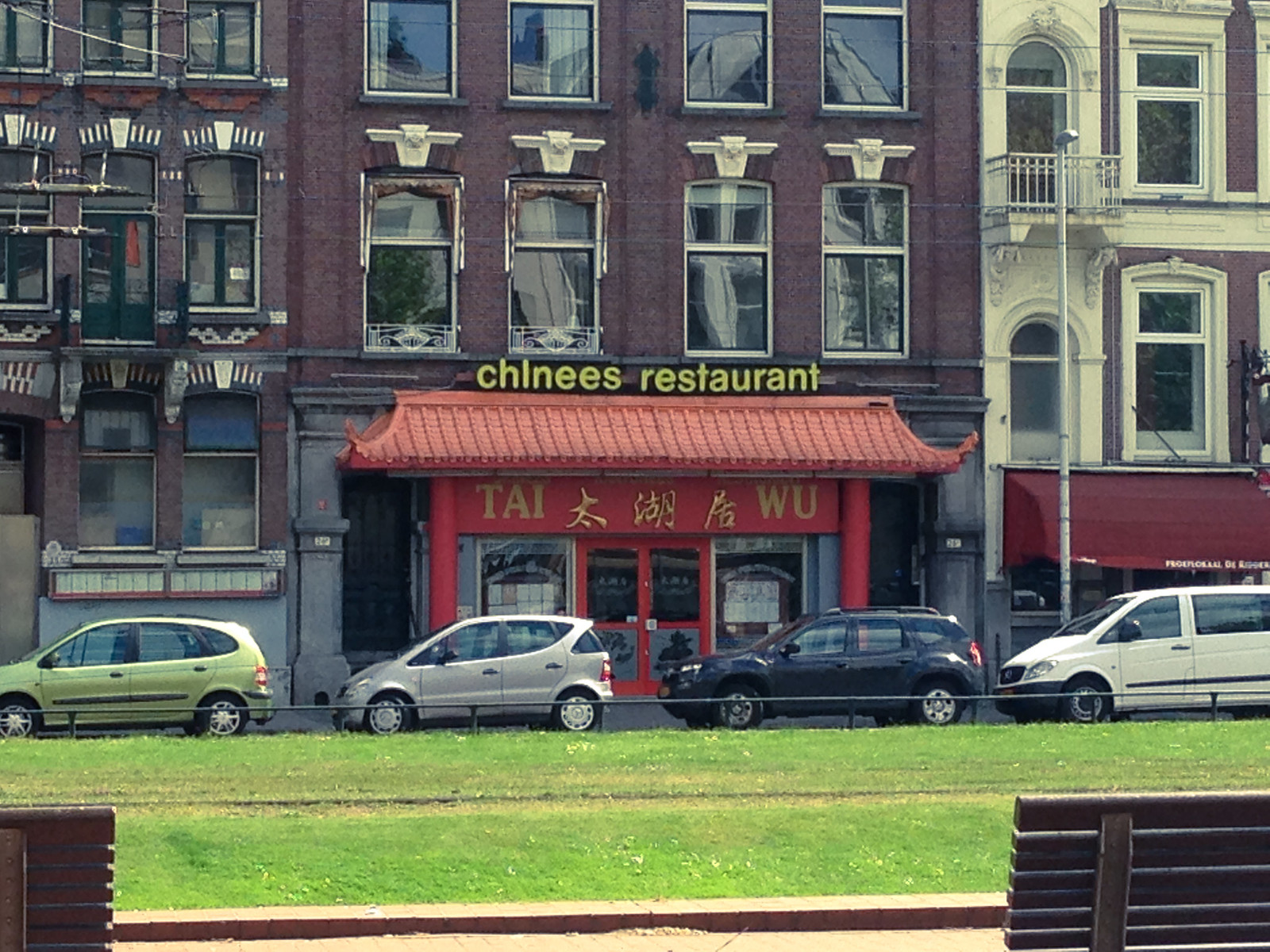The photograph captures a vibrant street scene in what appears to be a city like San Francisco, characterized by tall Victorian-style buildings. The central focus is a red-bricked Chinese restaurant named "Tai Wu," distinguishable by its ornate red facade and traditional Chinese architectural elements. On the roof of the first floor, the words "Chinese Restaurant" are displayed in yellow letters, albeit with a misspelling, reading "CHINEES." Between the words "Tai" and "Wu," Chinese characters are also visible. Above the restaurant, the building extends into several stories of what seem to be apartment units, containing rows of windows with decorative elements.

The street is lined with similar multi-story buildings, one to the left of "Tai Wu" with a simpler design and another to the right featuring white ornate window frames. In front of the restaurant, several cars including green, gray, black, and white are parked along the street. Directly across from the dining establishment, there is a small grassy area with two wooden park-style benches. The overall scene is lively and bustling, with a mix of architectural styles and urban greenery.